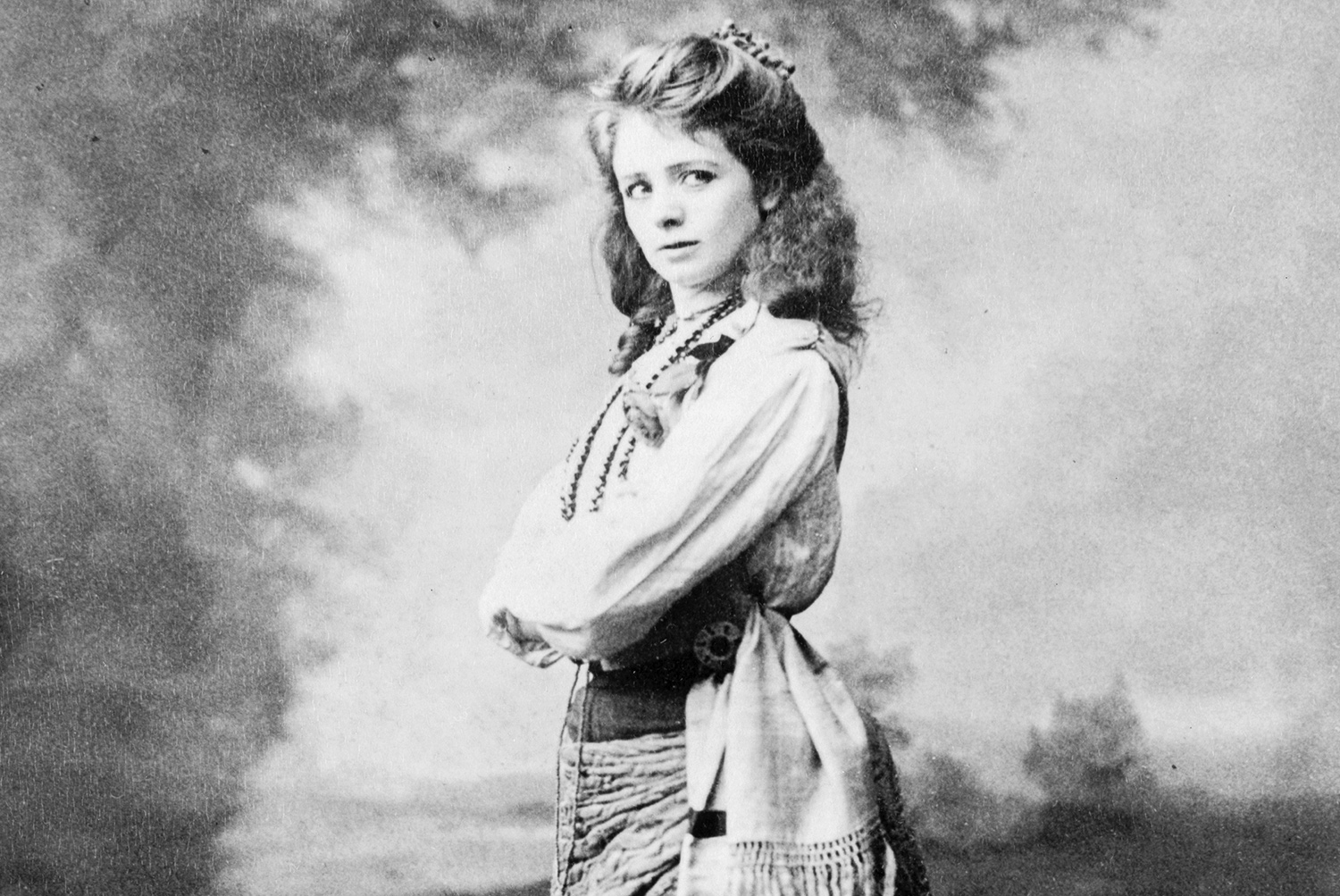This is an old black and white photograph, reminiscent of the Western times, likely from the late 1800s or early 1900s. The woman in the image is facing slightly to the left but appears to be looking upwards and to her right, with a curious expression. She has dark brown, frizzy, shoulder-length hair that is pulled back with a scrunchie. Her attire includes a dress or skirt paired with a long-sleeve shirt that is puffed at the sleeves and tucked into her dress, giving it a prairie-like or Native American appearance. A wrap or towel seems to be draped around her waist, and she is adorned with large necklaces and flowers draped around her neck. Her arms are crossed in front of her chest. The backdrop is blurred, featuring indistinct trees, with one tree covering the left half of the photo. This carefully composed image, evocative of scenes from books or movies about the Western era, captures her amidst a natural, albeit out-of-focus, setting.